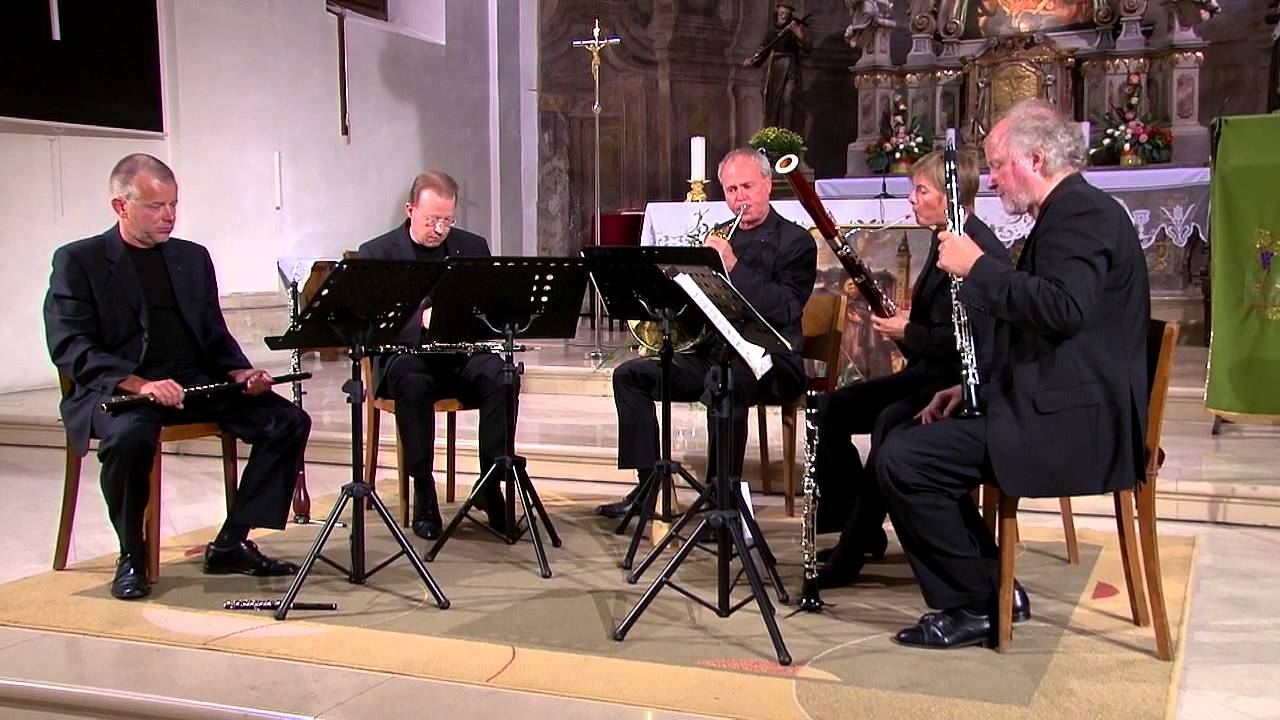This photograph captures a quintet of musicians, composed of four men and one woman, performing or rehearsing inside a beautifully ornate church, possibly Catholic as indicated by the religious iconography. The musicians, dressed in formal black attire including suit jackets, shirts, pants, socks, and shoes, are seated in a semicircle on wooden chairs positioned on a thin carpet with a yellow border and greenish-gray center, over a beige tile floor. Each musician has a black metal music stand with sheet music in front of them.

The group predominantly features woodwind instruments: the musician on the far left holds a clarinet, the next musician’s instrument is obscured by a stand, the middle musician is blowing into a brass instrument, the following musician is a woman playing a large bassoon, and the musician on the far right has what appears to be a clarinet with keys. Behind them, the church’s interior boasts a tall crucifix with a small statue of Jesus, set against a backdrop of stone columns and potentially a tabernacle with a large candle. The area is well-lit, showcasing the fine details of both the musicians and the elaborate architecture.